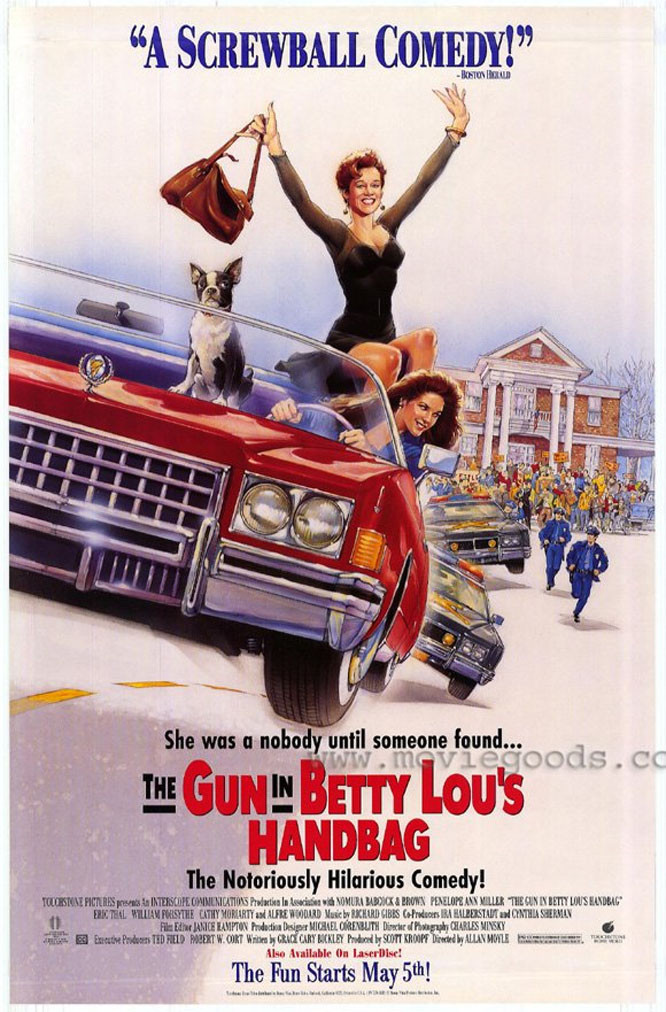The image is a detailed movie poster for the film "The Gun in Betty Lou's Handbag," described as "the notoriously hilarious comedy." The tagline reads: "She was a nobody until someone found the gun in Betty Lou's Handbag," with the premiere set for May 5th. The poster portrays a vivid scene featuring a bright red Cadillac convertible with a white background. 

At the top, a blue caption in all capital letters states, "A screwball comedy," attributed to the Boston Herald. The main visual shows a dark-haired woman driving the car, looking into the rearview mirror, accompanied by a small black and white Boston Terrier dog. A striking redhead, dressed in a tight, long-sleeved black dress accentuated with jewelry, sits on the trunk of the car, her feet inside the vehicle. She is holding a brown overnight bag in her raised right hand, appearing elated. 

The red Cadillac is being pursued by two police cars, with uniformed policemen and a crowd of spectators visible near a colonial-style brick building in the background. The chaotic yet humorous scene underscores the film's screwball nature. Additional smaller images on the poster make it busier, but the overall background remains predominantly white.